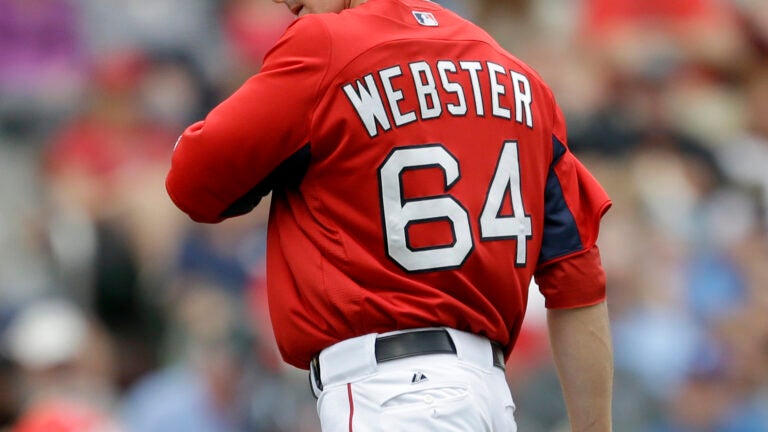This landscape-oriented photograph captures a baseball figure, possibly a manager, walking with an air of contemplation. The individual is wearing a red jersey with black accents, notably under the armpits, emblazoned with the name "Webster" and the number "64" in bright white font. The MLB logo is prominently displayed at the top of the collar. Their white pants, featuring a red stripe down the side and secured with a black belt, are cut off just below the top, giving way to a slightly bulky upper body, possibly puffed by the wind. Only a small portion of the person's mouth and right arm can be seen, while the hand is cut off from the frame. The colorful but out-of-focus background suggests a vibrant, busy crowd, adding depth to the scene.